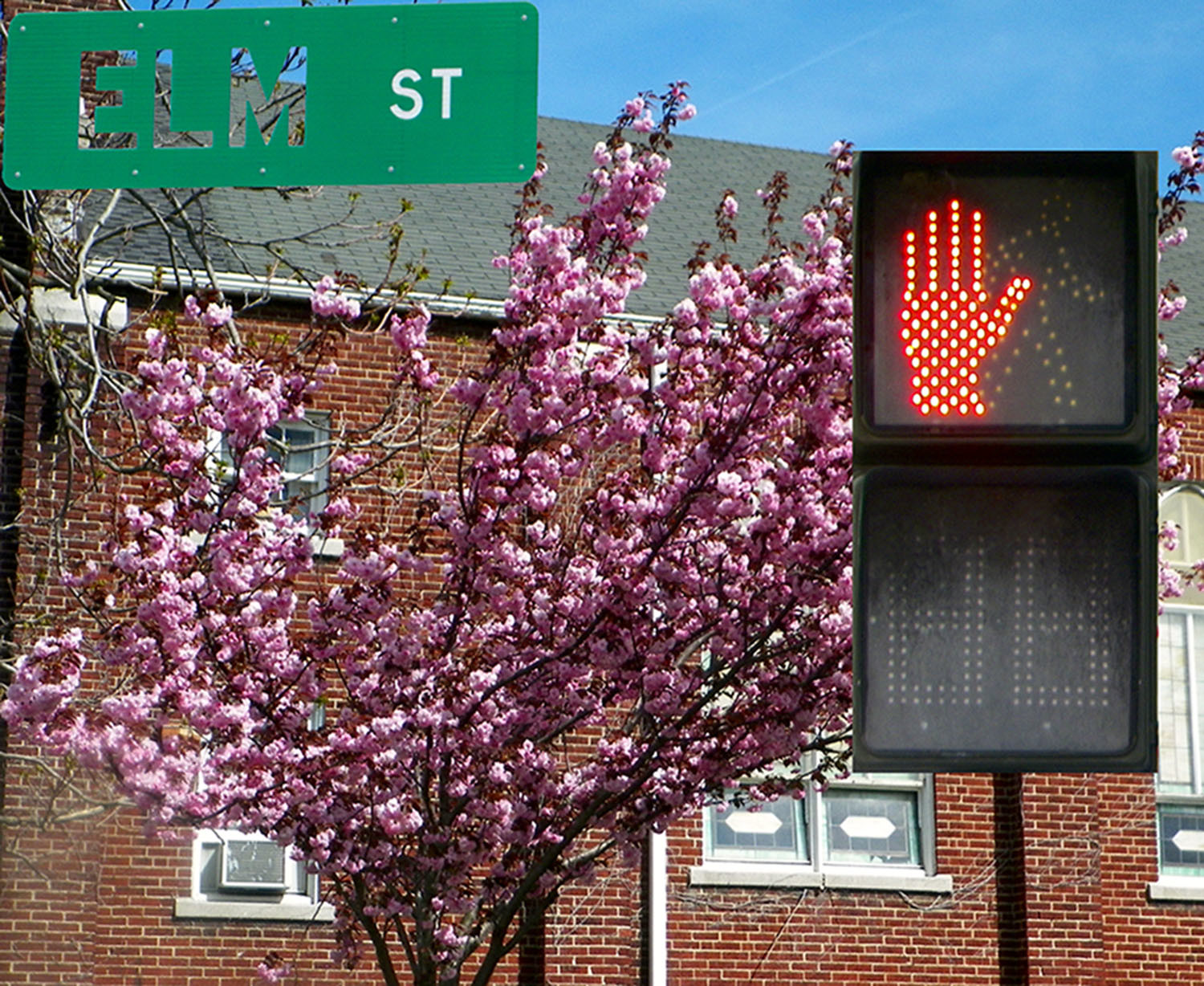This outdoor photograph captures a beautifully detailed street scene on Elm Street. Dominating the composition in the foreground, a vibrant cherry blossom tree is in full bloom, its pink and dark pink flowers reminiscent of cotton candy. Nestled behind the tree, there is a tall, brown-bricked building with at least two stories, complete with a shingled roof and an air conditioner protruding from one of its windows. At the top of the image, the sky is a bright robin's egg blue, streaked faintly by the trail of an airplane.

Prominently positioned on the right side of the image is a black "Walk/Don't Walk" sign, mounted on a metal pole. The upper panel of the sign displays a red lighted hand, signaling that pedestrians should not walk, while the lower panel remains unlit but shows the faint outline of a walking man and the digits used to count down the seconds. In the upper right corner, affixed to the pole, is a green street sign with cutout letters spelling Elm Street, accompanied by the white letters "ST." Together, these elements create a vibrant and intricate depiction of a serene moment on Elm Street.